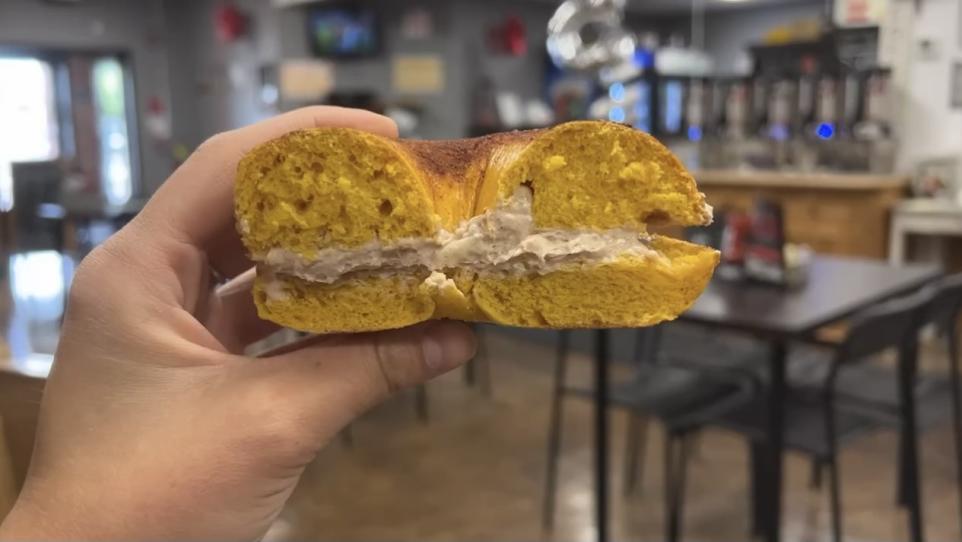In this close-up photograph taken indoors, the central focus is a person’s left hand holding a halved bagel sandwich. The bagel, which has a caramelized top and a yellowish hue, is filled with a mixture that appears to be tuna salad with mayonnaise, creating a creamy center. The background, though largely blurred, suggests the setting is a cafeteria or a diner-style restaurant. Visible in the background are square tables with chairs, a drink machine or soda bar, a TV, red fire alarms, and a front door with light filtering through. Some tables have condiment items such as ketchup and napkins, and the tiled floor can also be faintly discerned.